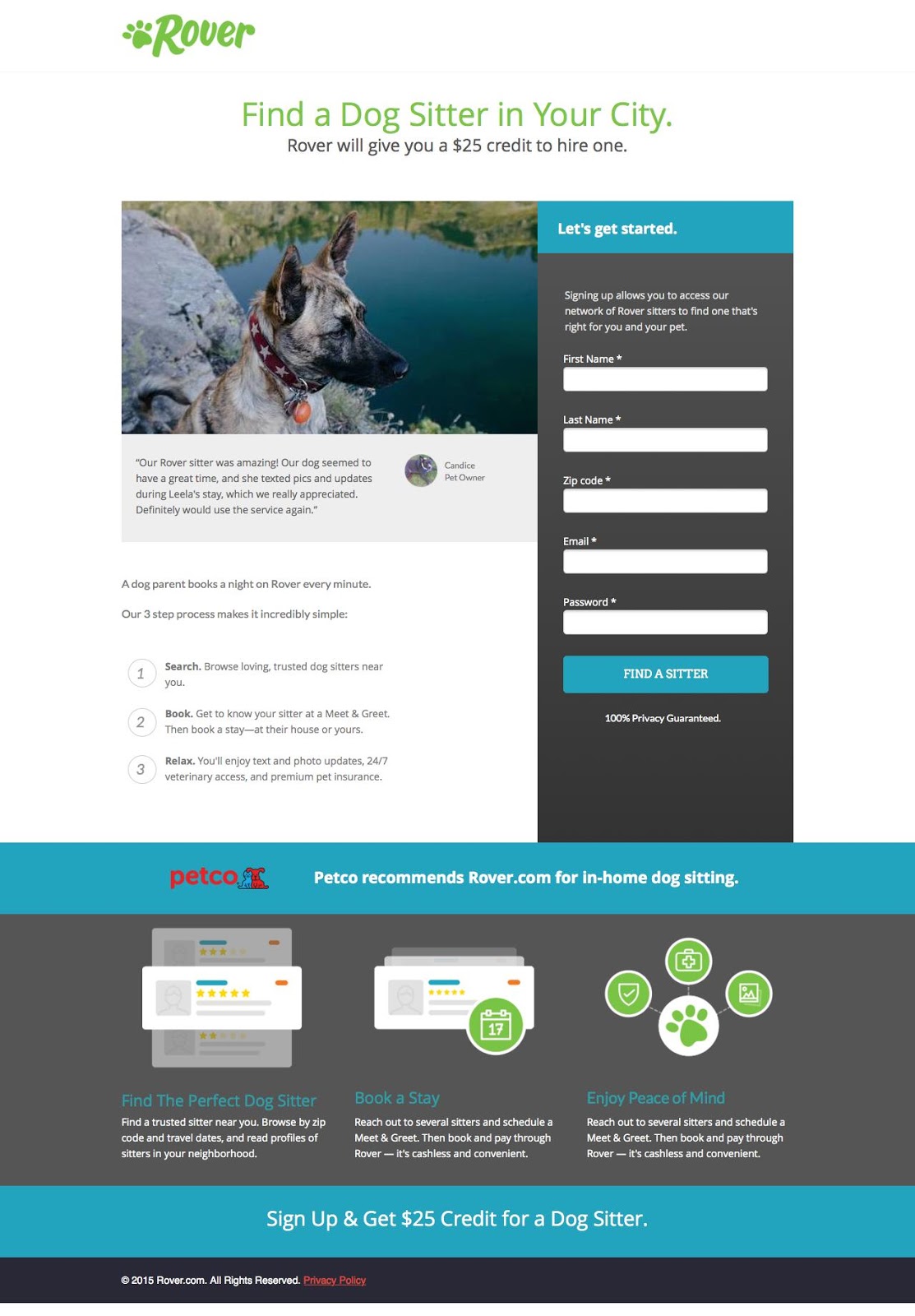This image is a screengrab from a webpage for Rover, prominently featuring branding elements at the top, including a dog's paw icon in green followed by the Rover logo. The middle section of the page includes a bold green header that reads "Find a dog sitter in your city." Below this, in black text, it mentions a $25 credit offered by Rover for hiring a dog sitter. The main visual element is a photograph of a dog sitting by a serene lake or pond, possibly accompanied by someone in camouflage, although only a part of this companion is visible, leaving room for ambiguity.

Further down, there's a testimonial section where a pet owner named Candice praises the Rover service, highlighting that their sitter was amazing, kept their dog happy, and provided regular updates and photos during their dog Leela's stay. This part is followed by a prominent call-to-action area on the side, inviting users to "get started" by entering their first name, last name, zip code, email, and password. This section features a teal-colored button labeled "Find a sitter." 

Towards the bottom of the image, the webpage emphasizes the ease of using Rover with a note that "a dog parent books a night on Rover every minute," and describes their straightforward three-step process: search, book, relax. The layout is clean and user-friendly, with various additional sections visible, supporting the main content.